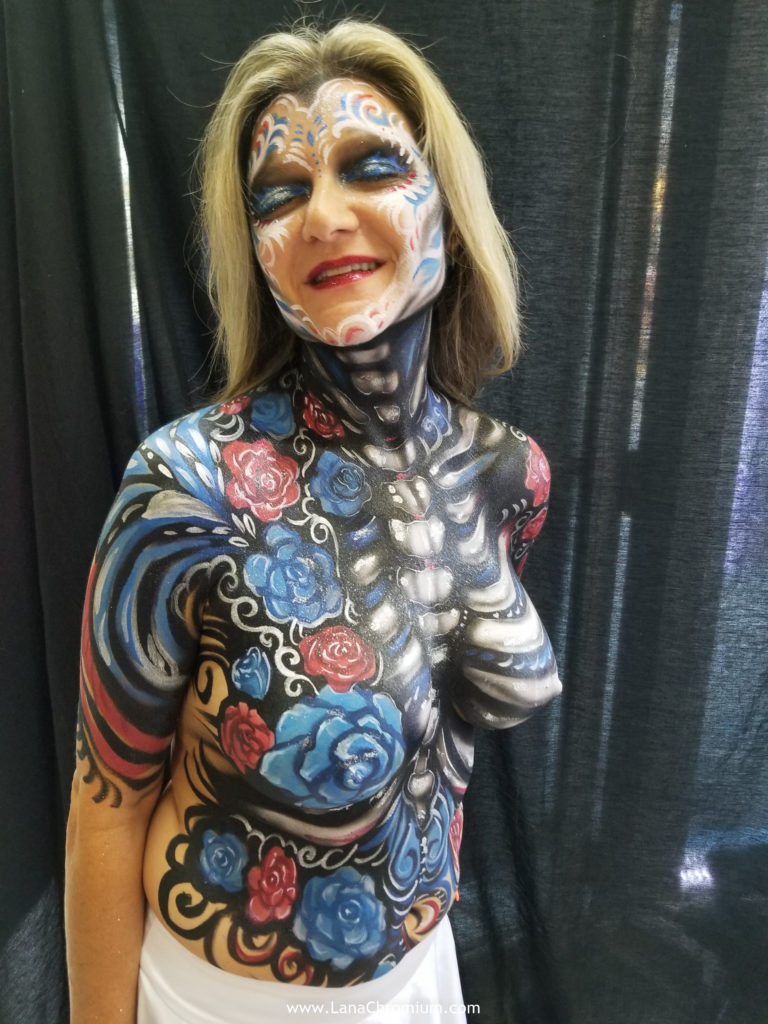This is a detailed photo of a woman in her mid to late 40s with shoulder-length, light brown to dark blonde hair, standing against a backdrop of black curtains with light filtering through. Her eyes are closed, and she is topless with intricate body paint covering her torso, breasts, abdomen, upper arms, and face. The body paint features a striking combination of blue, red, and white hues, forming a flowery design interspersed with swirls and a skeleton effect running down the center of her body, from her neck to her sternum and ribcage. Her face is adorned with red lipstick and designs reminiscent of a Mexican sugar skull, including blue paint across her eyelids and red and blue swirls. She is slightly turned, with her head tilted to the left. While her forearm remains unpainted, she wears white bottoms, and the text "www.moana, sheminium.com" can be seen at the bottom of the image.